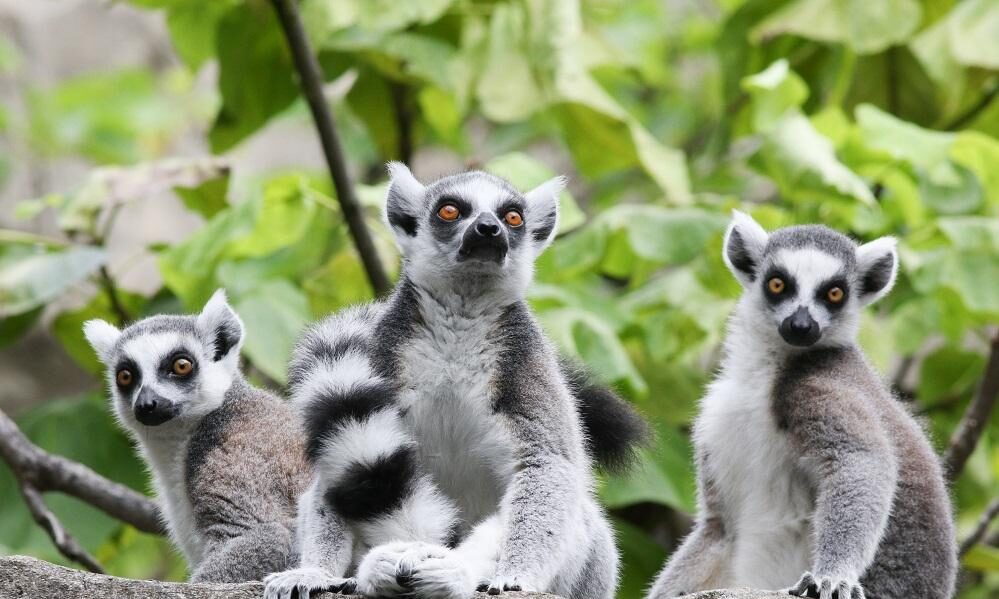In this daytime wildlife photograph, three lemurs are prominently featured against a backdrop of large, green plant leaves and tree branches. The lemurs, with their distinctive gray fur, have white chests, faces, and feet. Black fur encircles their striking orange eyes, which are wide open with black pupils, giving them a somewhat eerie appearance as they all gaze directly at the camera. Their black noses and ears, white on the outside and black within, complement their soft brown coats covering their backs and the tops of their shoulders and arms. The lemur in the center, slightly to the left, has its white-and-black banded tail wrapped around its body, while the tails of the lemurs on the left and right are not visible. Two tree branches crisscross below the center of the image, one extending from the bottom left to bottom right, and another is barely discernible behind the central lemur.